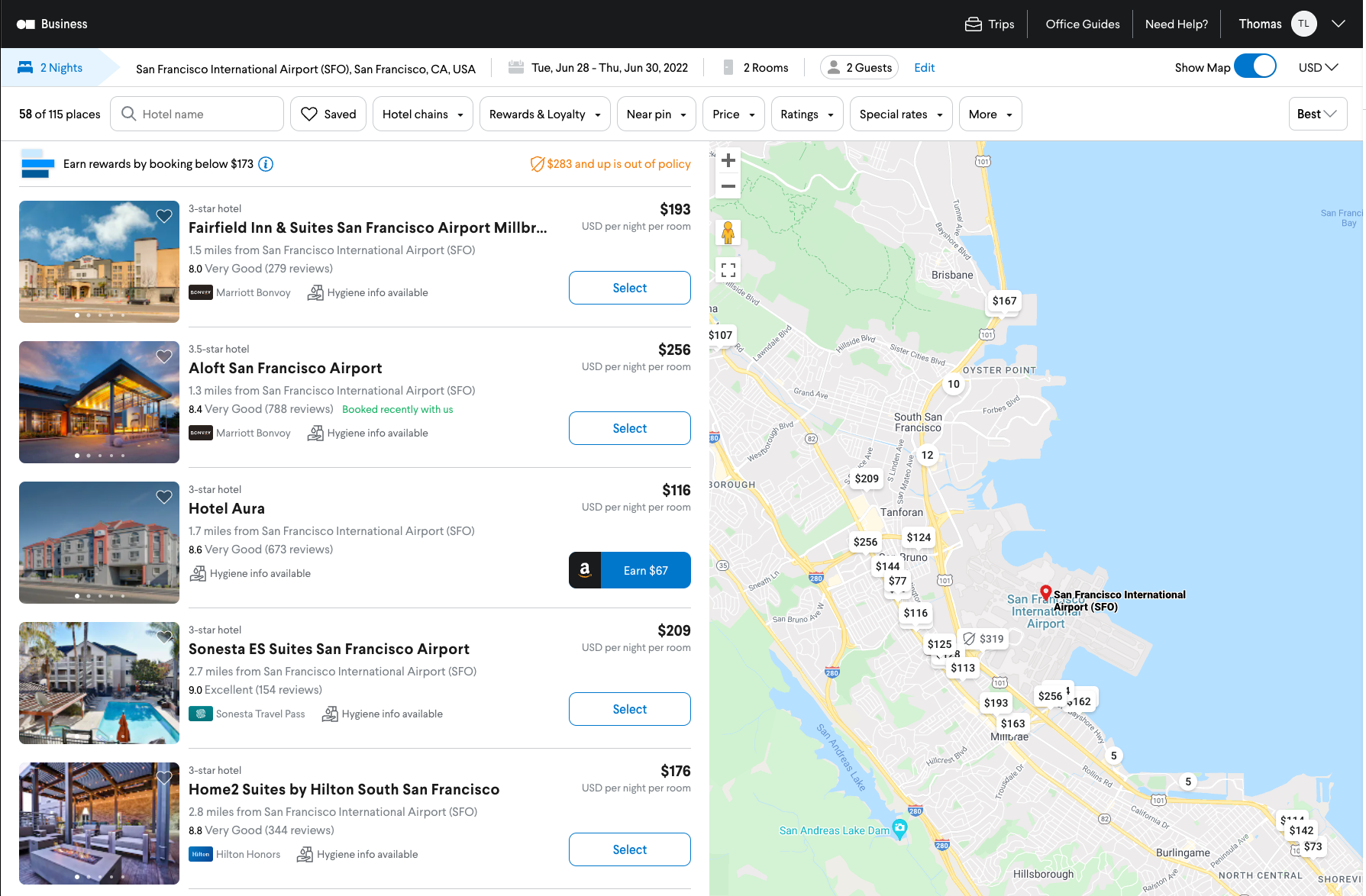The screenshot depicts a map and a selection of hotel listings near San Francisco International Airport (SFO), San Francisco, California, for a trip scheduled from Tuesday, June 28th to Thursday, June 30th, 2022. At the top of the screenshot is a black banner, where the upper left corner displays white text reading "Business." The right corner features options such as "Trips," "Office Guides," and "Need Help." The user's name, Thomas, is represented by the initials "TL" inside a white circle. 

The main content area begins with a search query for San Francisco International Airport followed by the specified travel dates and room requirements: "Two rooms, earn rewards by booking below $173." 

The first hotel listed is the Fairfield Inn and Suites, San Francisco Airport, priced at $193 USD per night per room. It is located 1.5 miles from San Francisco International Airport and has a rating of 8.0 ("Very Good") based on 279 reviews. To the left of this listing is an image of the hotel, which features tan, brown, and terracotta colors set against a blue and white sky.

The second hotel shown is the Aloft San Francisco Airport, a three-and-a-half-star accommodation, priced at $256 USD per night per room. It is situated 1.3 miles from San Francisco International Airport and has a rating of 8.4 ("Very Good") from 788 reviews.

The third hotel is Hotel Aura, a three-star property located 1.7 miles from San Francisco International Airport, with a rating of 8.6 ("Very Good") from 673 reviews, priced at $116 USD per night per room.